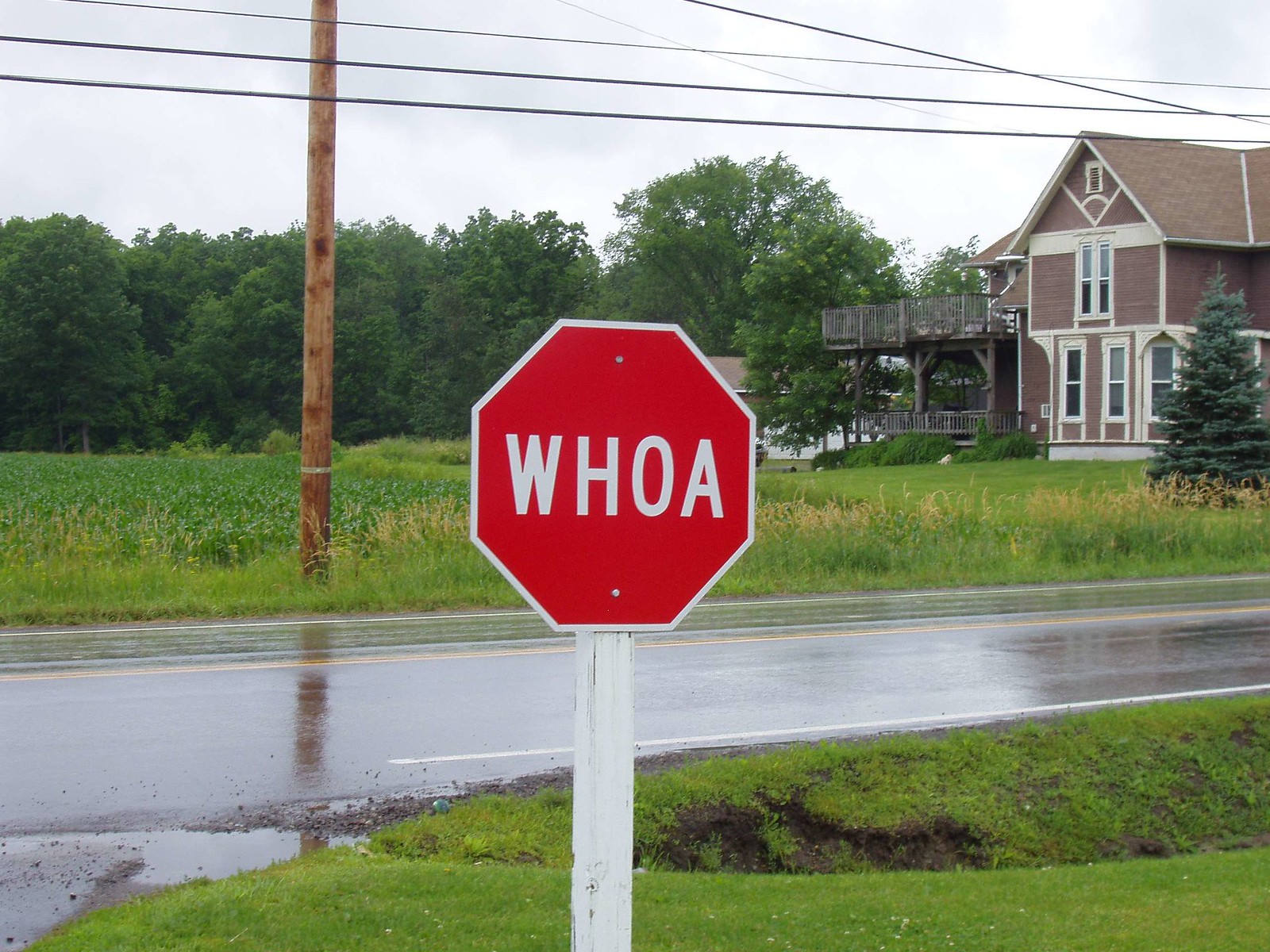This photograph captures a humorous homemade stop sign at the end of a driveway. The stop sign is affixed to a white post and bears the word "WHOA," adding a playful touch while still serving as a cautionary signal. The driveway itself is visibly wet, with puddles indicating recent rain and some noticeable erosion in the ditch alongside the nearby road. This road is a busier two-lane highway marked by yellow center stripes. 

Across the highway, a picturesque scene unfolds with a well-maintained lawn, a two-and-a-half-story home featuring two decks stacked on top of each other, and a row of old-growth trees including a prominent spruce tree. A cornfield stretches out beside the house, adding to the rural charm. Utility lines and poles are visible in the distance under an overcast sky, contributing to the sense of a recent downpour. The composition captures a blend of rural quirkiness and natural beauty, highlighted by the whimsical yet practical stop sign.